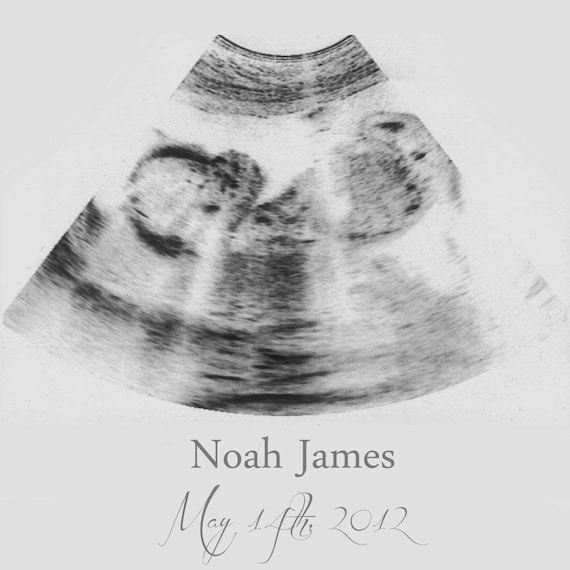The image is a detailed black and white ultrasound photograph, prominently displaying a side profile silhouette of a developing fetus. The ultrasound is situated against an off-white, light grey background. The fetus's head is discernible on the left side of the image, with part of the body visible on the right, resembling a nearly full-term baby. Beneath the vaguely U-shaped ultrasound image, the name "Noah James" is inscribed in bold, straight font, and the date "May 14, 2012" appears underneath in elegant calligraphic text.